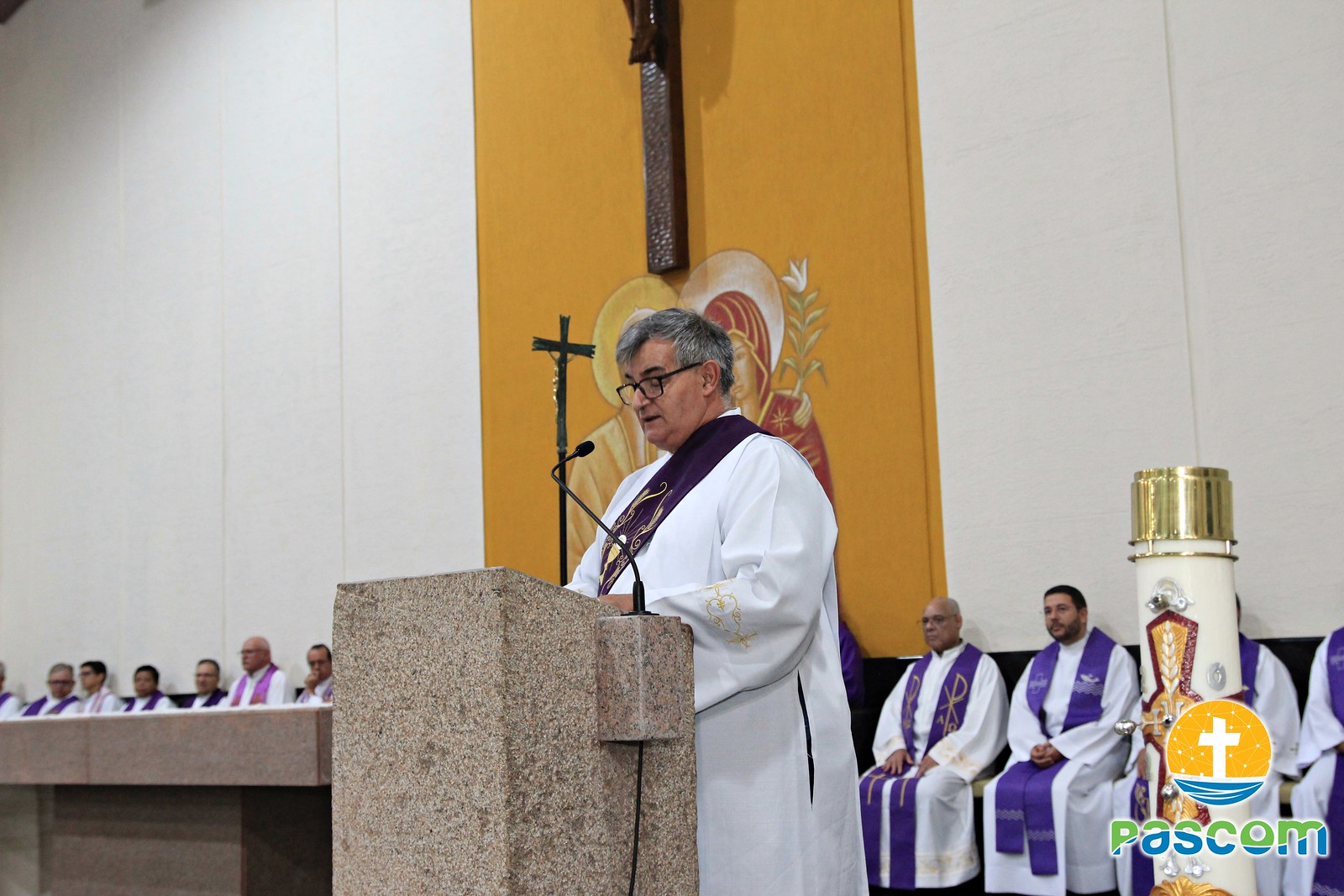The image is a detailed color photograph capturing a scene within a church, focusing on a priest or pastor standing at a light sandy brown podium. The priest, an older man with peppery gray hair and glasses, is adorned in a white robe and a purple stole. He speaks into a small black microphone positioned at the podium's edge. Behind him, several other clergymen are seated, all dressed similarly in white robes with purple stoles of varying shades. The background features a striking gold horizontal stripe on the wall, partially obscuring a large wooden cross with the lower part of Jesus' legs visible. Additional religious images are partially blocked by the speaker. The wall itself is primarily composed of white panels. In the bottom right corner of the image, a round logo with a white cross inside and the letters "P-A-S-C-O-M" in green and blue can be seen. The overall style of the photograph is realistic and representational, emphasizing the solemn and serene atmosphere of the scene.